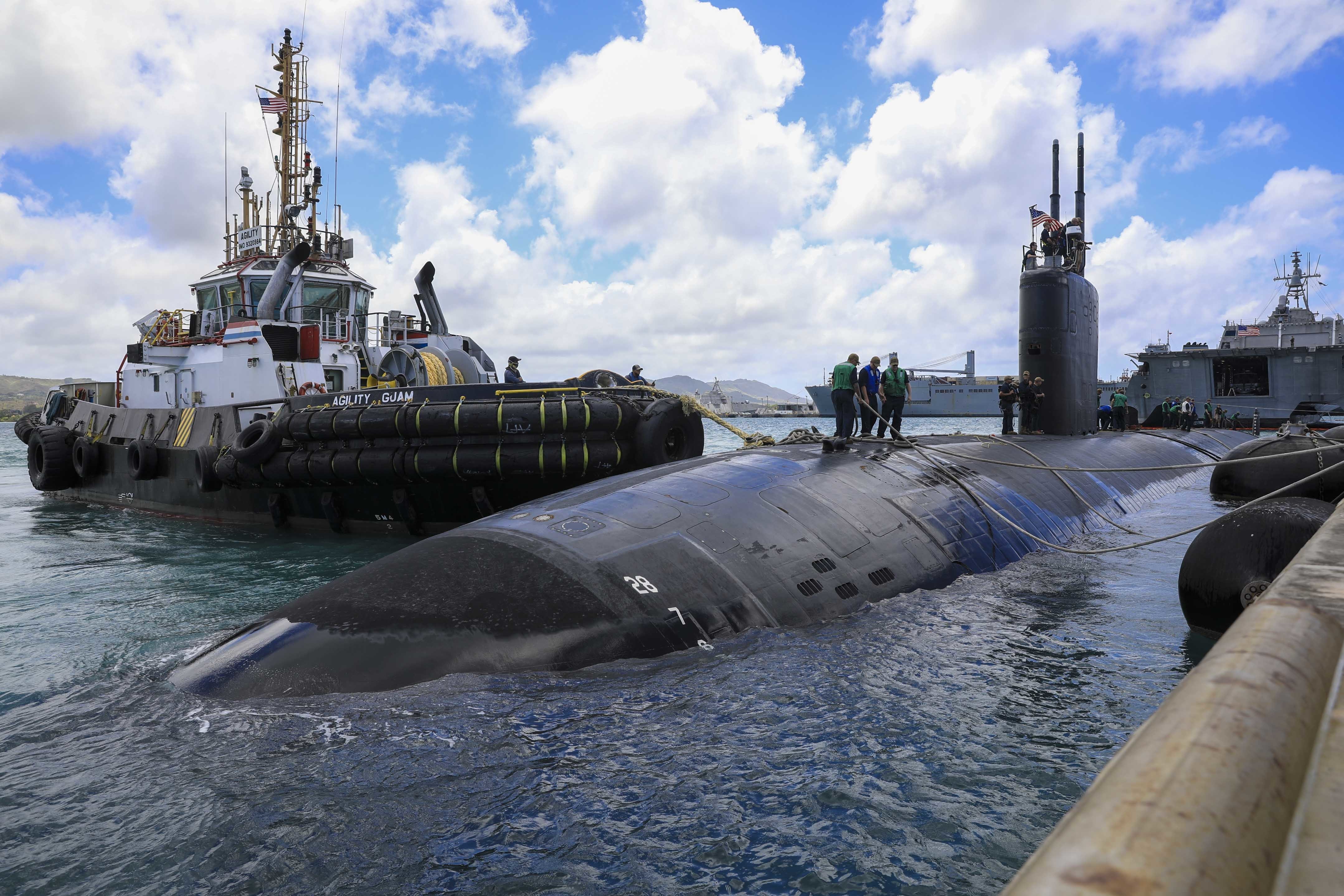In the vibrant seascape of daytime, a striking scene unfolds with a black submarine prominently positioned at the center of the image, floating above the water's surface. Atop the submarine, three men clad in black trousers and life jackets—two in green stationed at the ends and one in blue nestled in the middle—can be seen, presumably conducting maintenance work. The submarine proudly displays the United States flag atop its conning tower. To the left, a black tugboat with white highlights, labeled "Agility Guam," equipped with rubber tires for tugging, stands ready. Behind the submarine, a grey boat partially visible, is overshadowed by a larger aircraft carrier in the distance. The expansive sky above showcases a tapestry of white clouds interspersed with patches of blue, completing this bustling maritime tableau.